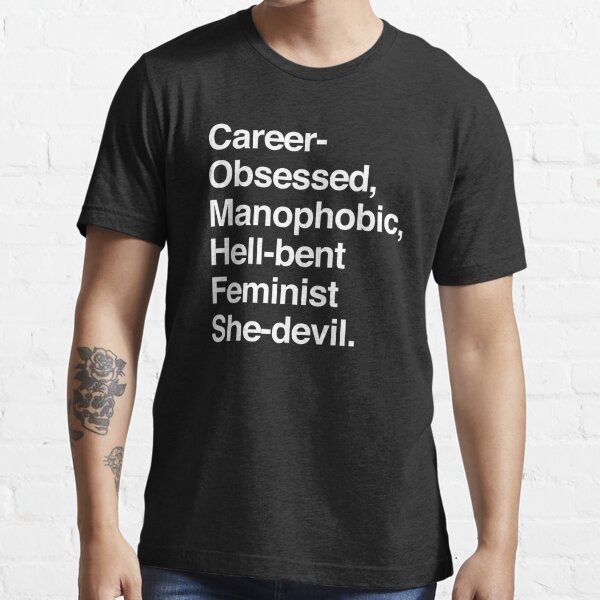A Caucasian man is pictured from the neck down, standing against a white background. He is dressed in a well-fitted, unwrinkled black t-shirt with white lettering. The text on the t-shirt reads: "career-obsessed, manaphobic, hell-bent, feminist, she-devil." He is also wearing blue jeans. The man has a noticeable tattoo on his right forearm featuring a black-outlined skull with a rose on top and black leaves extending from it. There is a second tattoo on his wrist, but its details cannot be clearly identified.